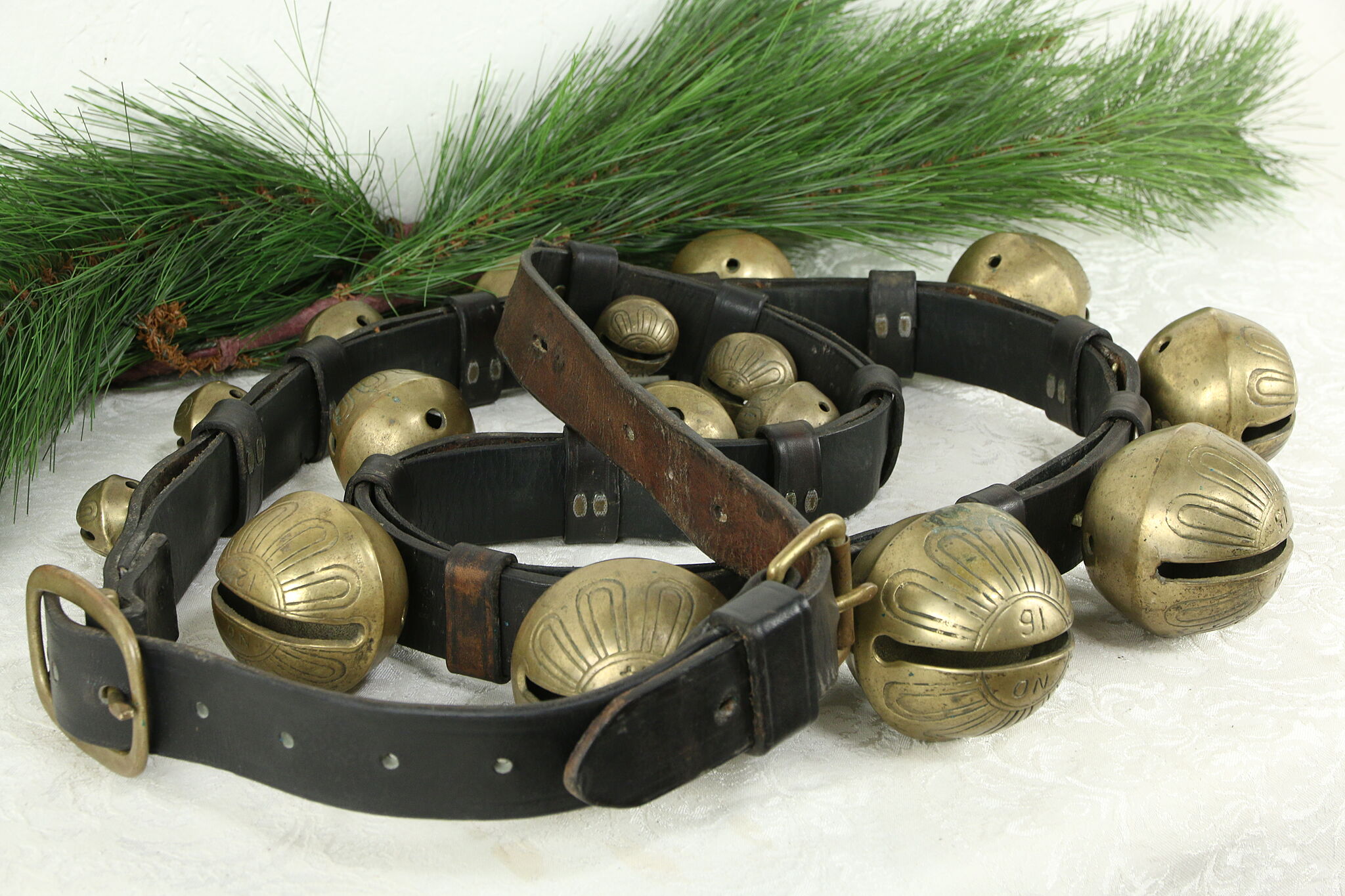The image displays a close-up of a unique Christmas decoration featuring a large, black leather belt adorned with an array of attached brass bells. The belt is composed of multiple segments joined together, showcasing a mix of small and large brass bells circling its perimeter. Two brass buckles are present: one square-shaped and another with an unconventional design, indicating it might be a combination of two belts. The belt, with a brown interior, rests in a somewhat heaped arrangement on a white cloth background. Flanking the belt are two sprigs of vibrant, long, and softly flowing green pine needles, adding a festive, seasonal touch to the intricate decoration.